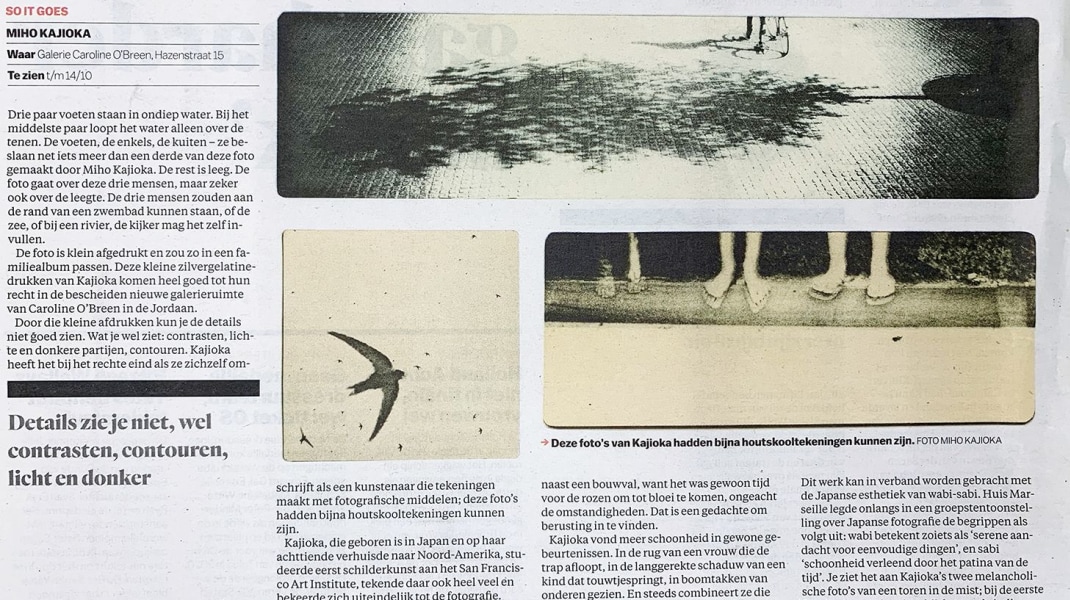The image is a clipping from a magazine or newspaper, characterized by black, white, and gray tones, with hints of red and tan. Dominating the left side, in red letters at the top, it says "So It Goes," followed by a mix of black-text details and multiple paragraphs in a foreign language, possibly Swedish, Dutch, or Russian. Among the text, some recognizable words include "Miho Kajoka" and "Ware, Gallery." The right-hand side features a long banner at the top that appears to be a photograph of the ground with a shadow cast on it. Below this banner, there's a striking black and white image of a bird in flight. Next to the bird, another image shows the feet of a couple of people standing side by side, possibly on a wooden plank. The overall layout and style of the text and imagery suggest that this was part of a structured, well-designed article typical of a magazine or newspaper page.